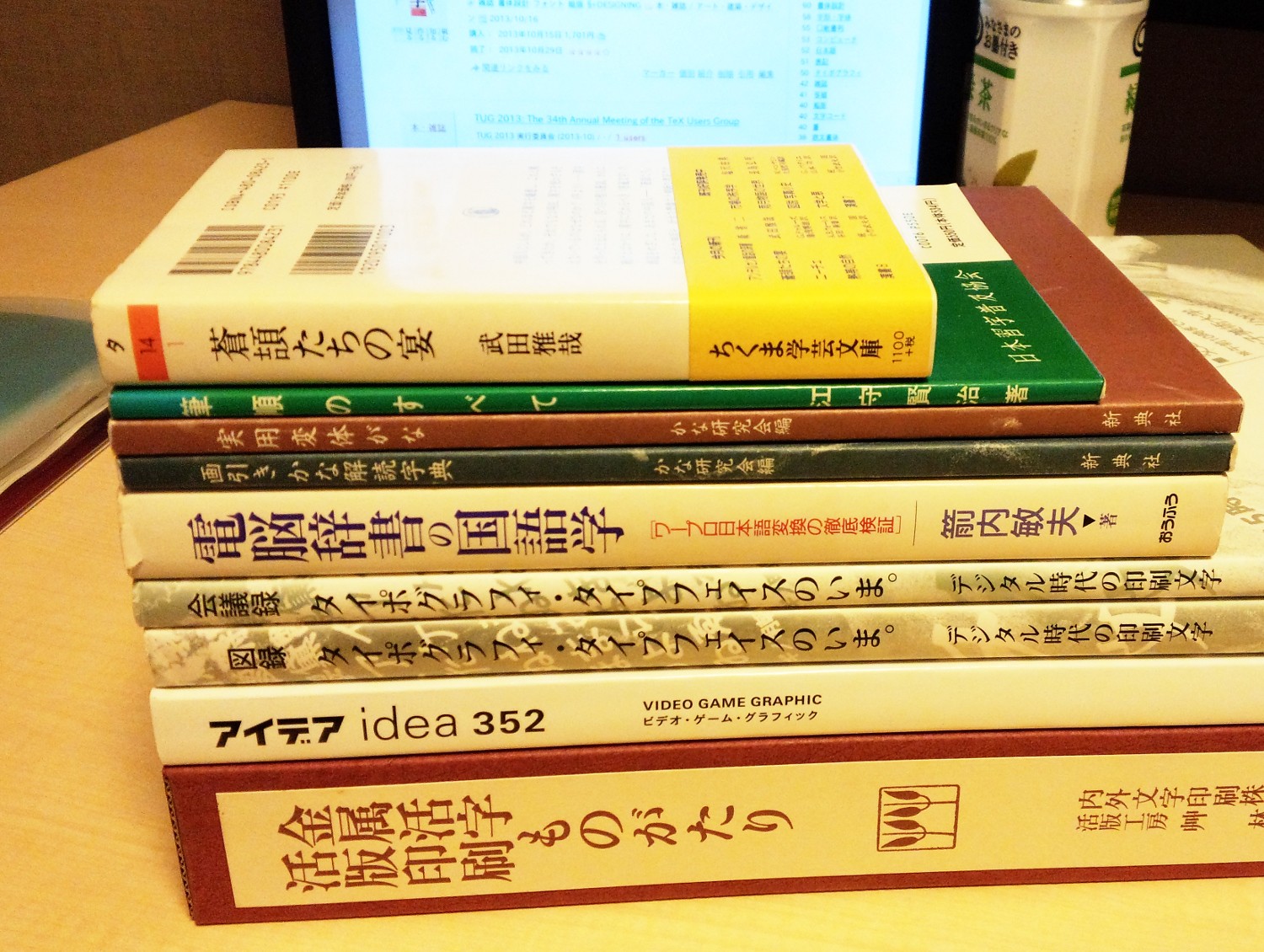This indoor scene, bathed in warm, orange-yellow lighting, features a meticulously aligned stack of books resting on a yellow table. The spines of the books, oriented perpendicularly to the camera, display various types of oriental writing, likely Japanese. From the bottom to the top, the stack includes a thick, large beige book trimmed in red with red oriental writing, and a second beige book that reads "VIDEO GAME GRAPHIC" along with "IDEA 352" in purple letters. Among the more colorful volumes, there is a thin green softcover with gold writing, and a beige and yellow hardcover with brown lettering. Two identical thin beige hardcovers with gray print and purple oriental writing are also part of the stack. In the background, a black computer screen is turned on, adding more modern elements to the image which also includes a white carton and a white cup with a leaf imprint and a cover beside the computer.